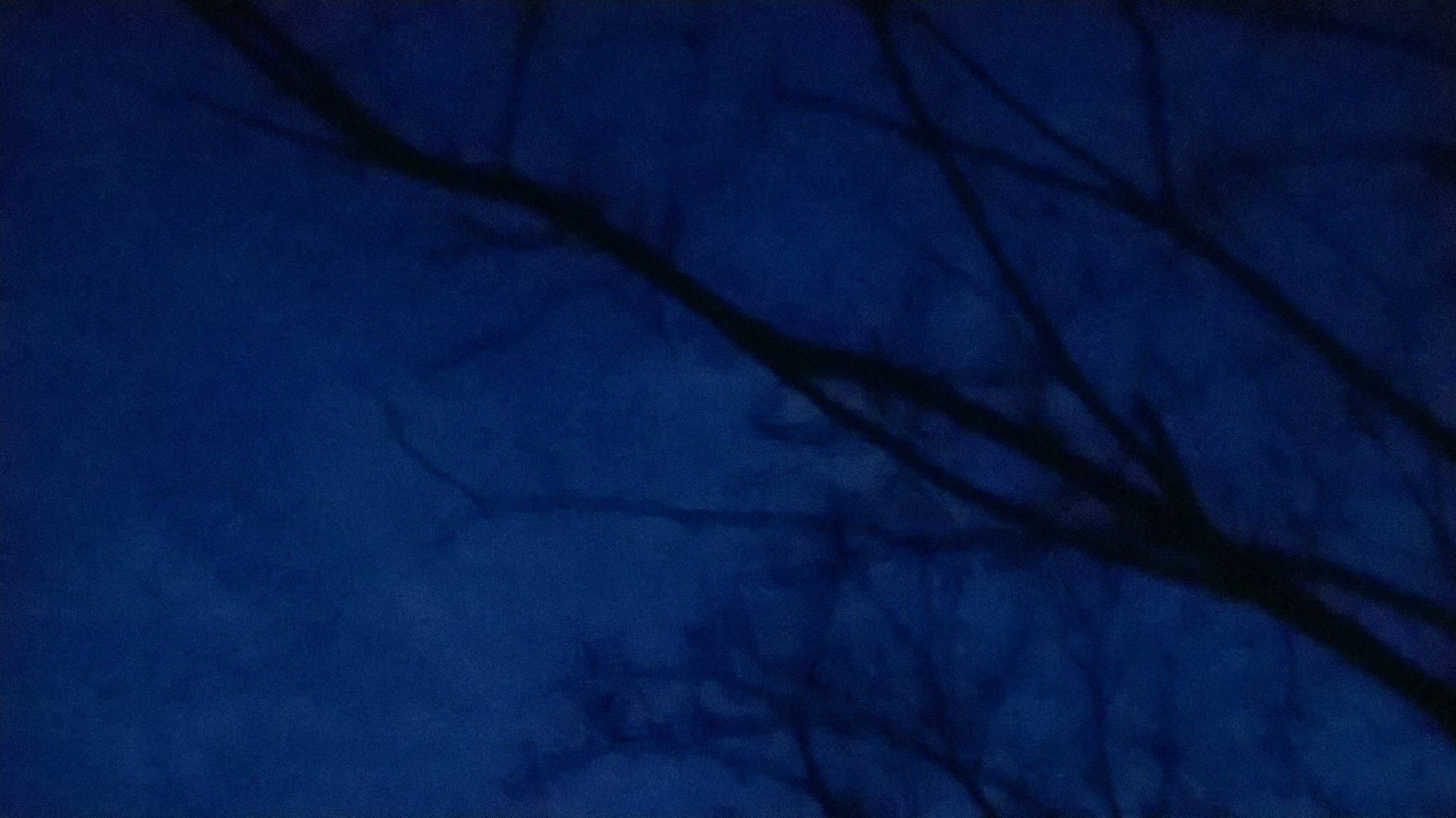A captivating and atmospheric horizontal photograph features a foreboding yet mesmerizing dark purple sky, transitioning to a lighter purple and magenta hue towards the lower half of the frame. Bare branches extend from the right and bottom right corners, reaching upward and out of the frame, their stark darkness contrasting sharply against the vivid sky. This eerie yet striking image, with its branches devoid of leaves, invokes a somber, mysterious mood, perfectly capturing a blend of nature's simplicity and dramatic color palette. The longer width compared to height underscores its horizontal orientation, creating a panoramic view of this hauntingly beautiful scene.